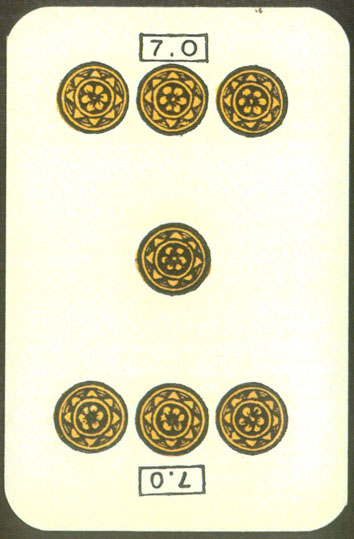This detailed illustration appears to be a tarot card. The card boasts a structured design, bordered by black corners against a yellowish-white background. Centered at the top and bottom of the card, a black rectangle houses the number "7.0," which is also repeated at the bottom in an upside-down fashion for symmetry.

Strategically placed across the card are seven intricately designed gold objects. Arranged with three at the top, one in the middle, and three near the bottom, these objects feature an elaborate floral design. Each object comprises an outer edge that transitions into petal-like forms, culminating in an innermost circle resembling a flower shape. 

The portrait orientation of the card, taller than it is wide, and the absence of any text beyond the numerical inscriptions, keep the focus solely on the geometric and aesthetic elements of the gold objects. Interestingly, the illustration is devoid of any human, animal, or plant imagery, staying true to its purely graphic representation.